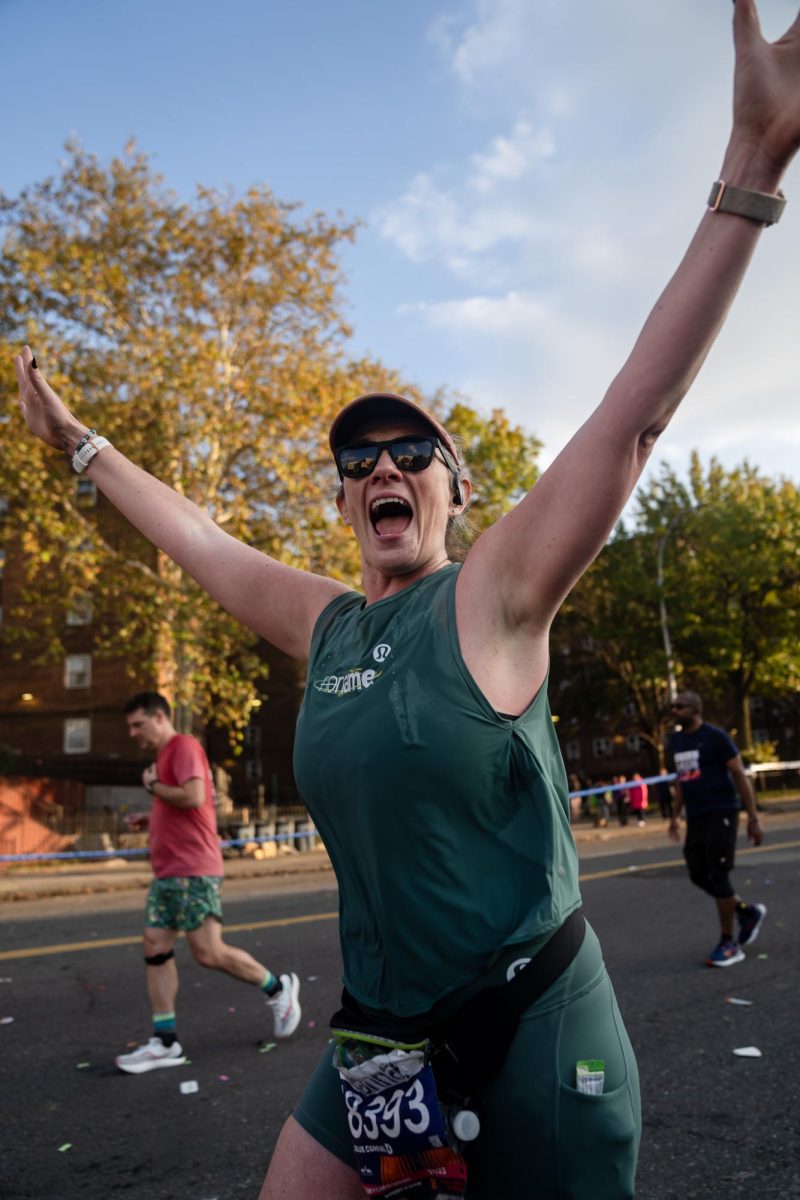The image captures a jubilant woman running down a dark gray asphalt road with a triumphant expression on her face. She has her arms raised in a V-shape, hands facing outwards, and her mouth wide open, revealing her excitement. She's dressed in a green tank top with white lettering across the chest, green shorts, and a visor paired with dark sunglasses. A black bag with the number 8393 is fastened to her waist. She wears a white watch on her left wrist and a gray-banded watch on her right wrist. 

Behind her, two other runners are also on the road. To her left, partially under her arm, a man in a red shirt, green print shorts, and white shoes can be seen, with a black band just below his knee. On her right, another runner dressed entirely in black, including his shirt, shorts, and shoes, follows with his arms down by his sides. 

The setting features a blue sky adorned with gray and white clouds towards the right. A tree with yellow leaves stands in the background, hinting at an autumn scene. The road is scattered with confetti, and a yellow line runs along the far side of the pavement. In the distance, additional trees and possibly a park can be observed, suggesting a communal and scenic marathon or running event.